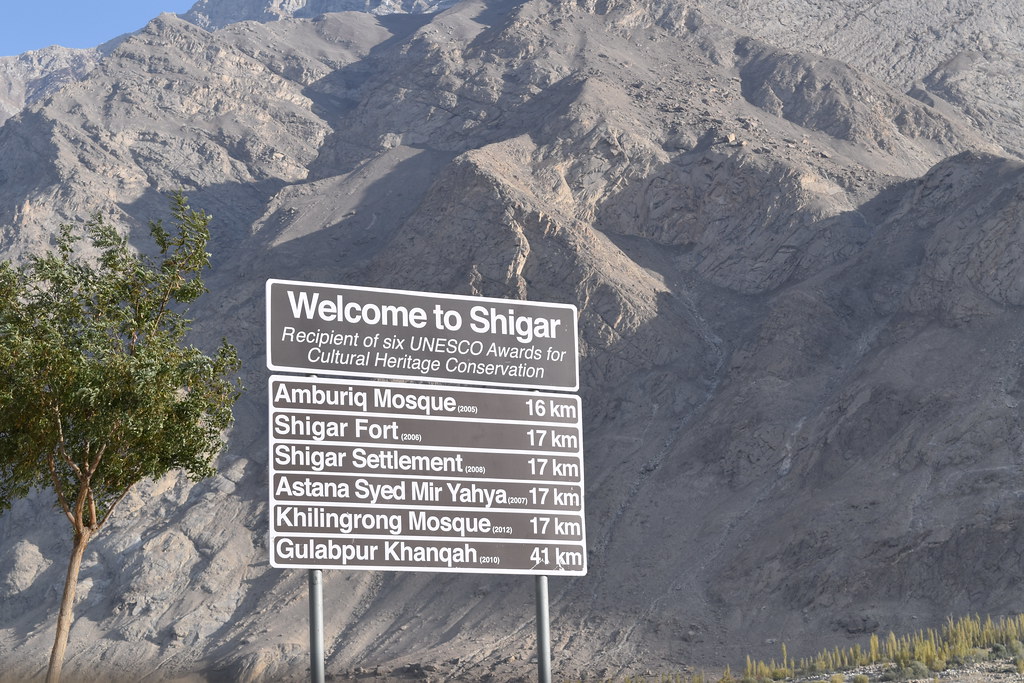The image captures a vast rocky mountain dominating the background, with its ash-gray, barren surface stretching across most of the composition. A sliver of blue sky peeks out from the top left corner, contrasting the rugged texture of the mountain. In the bottom left corner stands a single small tree with green leaves, providing a splash of color amidst the grayscale rocky landscape. At the center of the image, a large sign features prominently. The top part of the sign reads, "Welcome to Shigar, recipient of six UNESCO Awards for Cultural Heritage Conservation" in white sans serif letters. Below, it lists distances to various locations: Ambarik Mosque, 16 kilometers; Shigar Fort, 17 kilometers; Shigar Settlement, 17 kilometers; Astana Syed Mir Yaha, 17 kilometers; Killingrong Mosque, 17 kilometers; and Gulabpur Kangkwak, 41 kilometers. The scene is an outdoor capture, emphasizing the contrast between the massive rocky background and the solitary tree and informational sign in the foreground.